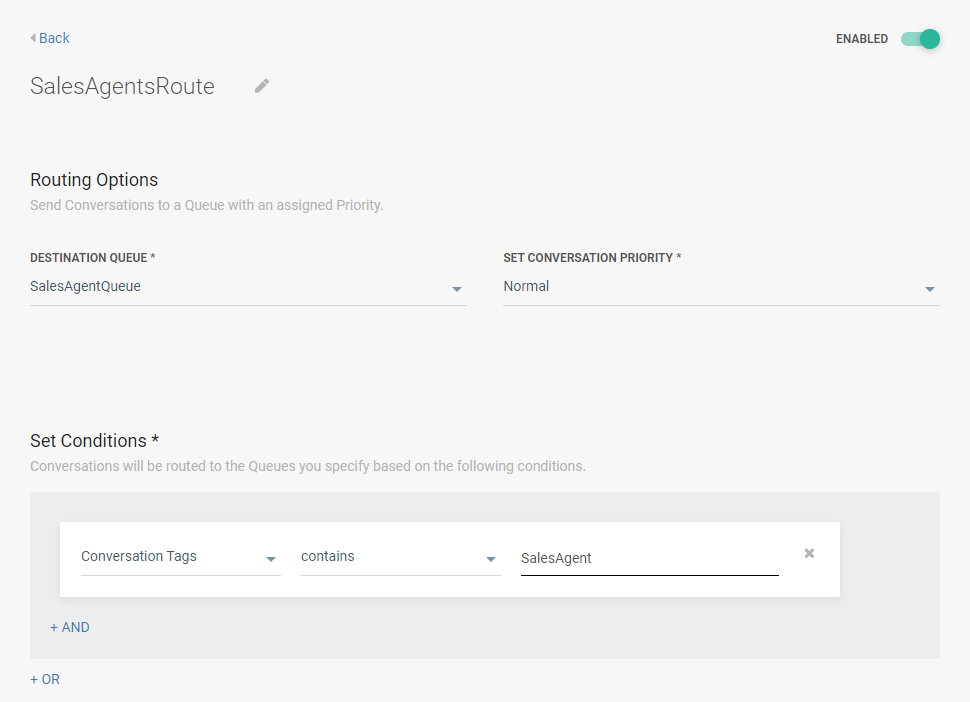The screen displays an interface with a light gray background titled "Sales Agents Route" at the top. In the upper right-hand corner, there is a toggle switch labeled "On/Off," which is currently set to "On." The interface appears to be a dashboard for setting routing options for sales conversations. It features sections for configuring various parameters. 

The primary heading "Sales Agents Route" is reiterated beneath the title, followed by an explanation that reads "Routing options in conversations to a queue with an assigned priority." 

Several interactive fields are visible: one to "Select a Destination Queue," another to "Set Conversation Priority," and a section at the bottom titled "Set Conditions." This section stipulates that conversations will be routed to the specified queues based on certain conditions. It appears to be a tool designed for managing and prioritizing sales-related conversations, possibly for the purposes of customer support or sales management within a computer program, website, or application interface.